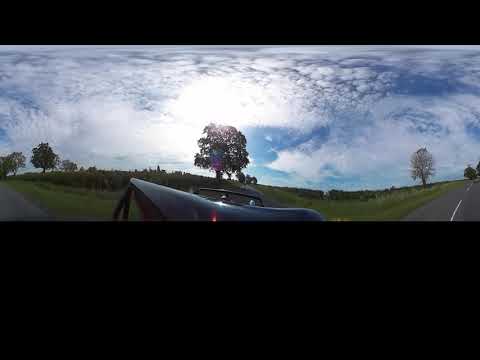The image is a panoramic outdoor view with a significant focus on the sky, characterized by a combination of deeper blue hues and a dense layer of light white clouds. The sun, though obscured by the clouds, creates a luminous effect on the surroundings. The landscape is dominated by a large tree centrally located in the distance, surrounded by a grass-covered field interspersed with either small trees, lower bushes, or darker tall grass. The image appears to have been taken from a road, which is visible both on the left and right, each stretching diagonally and converging towards the center, giving the scene a warped, curved effect consistent with a 360-degree camera perspective. The foreground includes a reflective surface—possibly part of a car dashboard or open car door—adding to the distorted panorama. Additionally, the photograph is framed by black bars along the top and bottom, with the lower bar occupying about one-third of the image, contributing to the overall dramatic presentation of the scene.